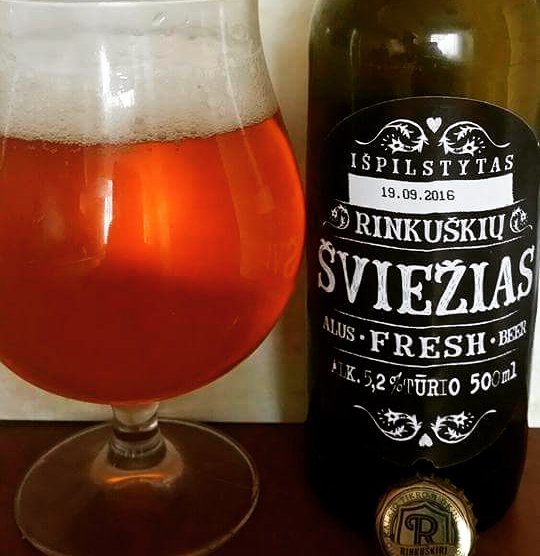The image depicts a rich amber-colored beer with a foamy head about an inch tall, served in a teardrop-shaped glass on the left side. The glass is three-quarters filled, sitting upright on a surface with a white backdrop, suggesting an indoor setting with appropriate lighting. Next to it, on the right, is a dark-colored, olive green bottle, adorned with a black label featuring intricate designs—tiny white hearts, curly leaves, and flowers. The bottle label includes text in a foreign language, likely Slovakian, with prominent English words "fresh" and "beer." It notes an alcohol content of 5.2 percent. The bottle, with a gold seal at the bottom, also has the term "Ispilstytas," and an expiry date of September 19, 2016.